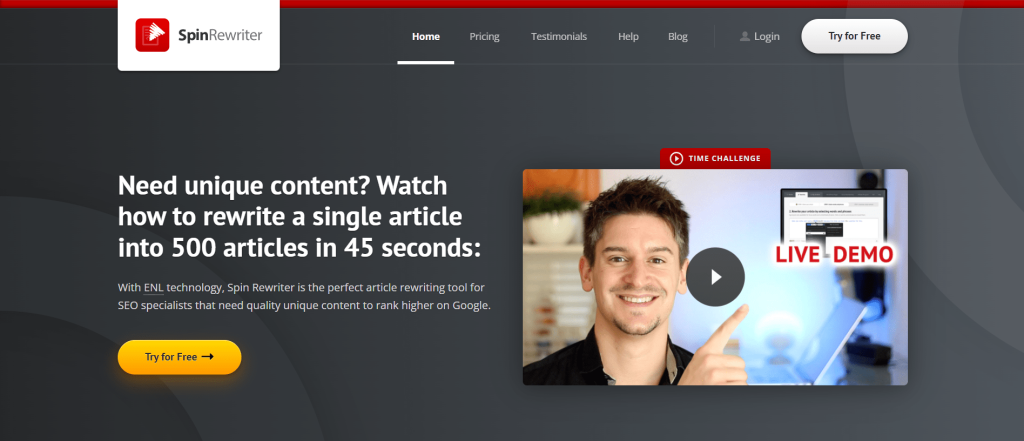In this image, we are looking at a screenshot of an online website interface set against a dark gray and black background. The design features two geometrical gray shapes, a half circle in the upper right corner and another in the lower left corner. A thin red border stretches from the upper left to the upper right corner. Below this border, centered in white text, are navigation links: "Home" (which is underlined, indicating the current page), "Pricing," "Testimonials," "Help," "Blog," and "Login." 

In the upper left corner of the screenshot, there's a white box containing a red and white logo to the left, and to its right, the company name "Spin Rewriter" is displayed. The upper right corner features a prominent white action button with "Try for free" written in black text.

On the right side of the image, there is a video screen with a play button overlay. The person visible on the screen appears to be a Caucasian man around 30 years old, sporting a mustache and a thin beard, and wearing a black collared shirt. His right hand is visible, pointing upwards toward another smaller screen within the main image. This smaller inset reads "Live Demo" in red text. Above it, there is a small box with the label "Time Challenge."